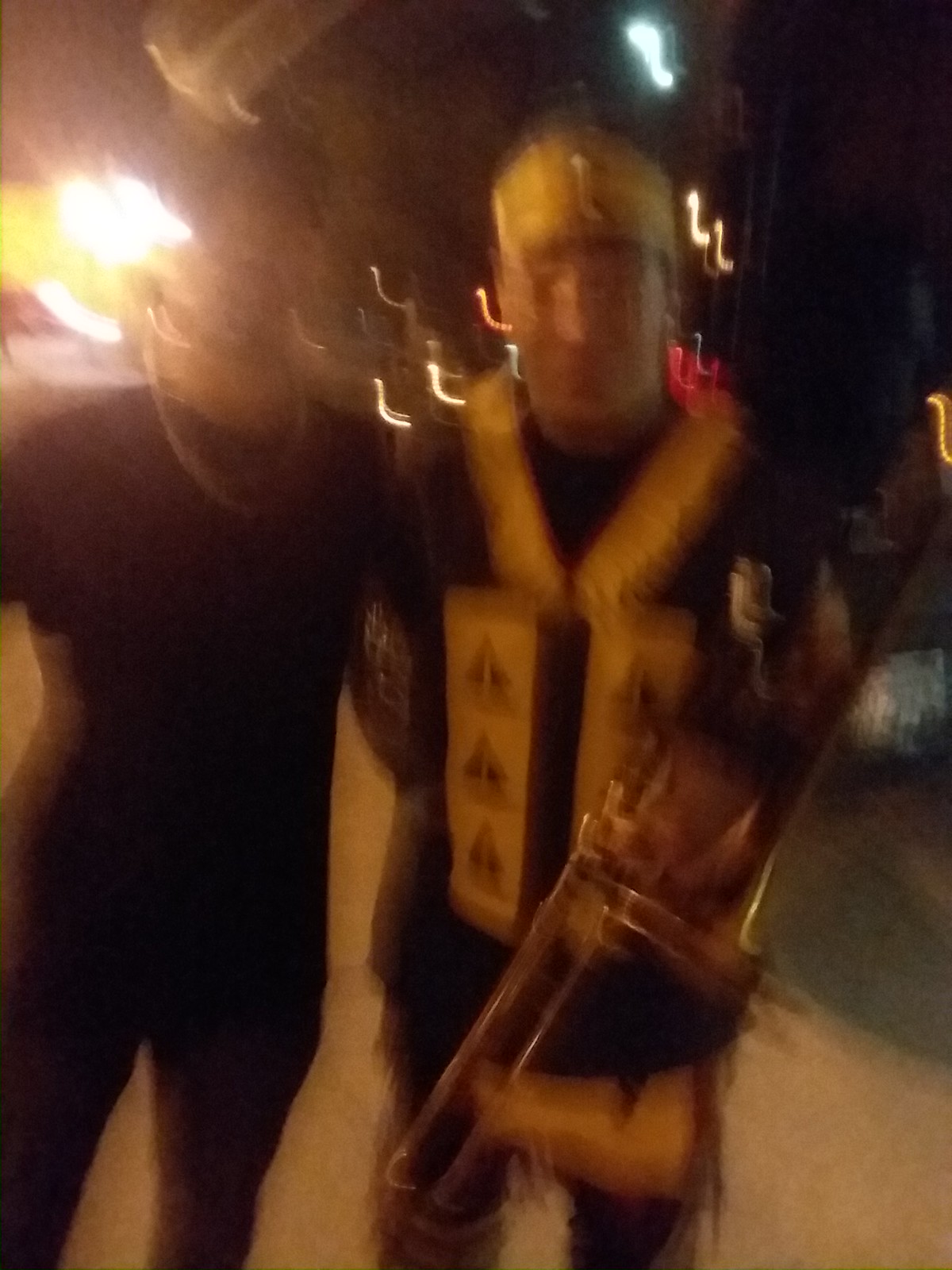In the photo, captured at night, two figures are seen standing outside under a bright light source in the top left corner, which casts a strong glow against the backdrop. Though the image is blurry, it appears that these individuals could be actors wearing elaborate costumes. The figure on the right wears a unique golden hat with a shape resembling an "L" and is dressed in a distinctive ensemble: a black vest accented with a golden collar and two hanging golden pieces adorned with triangles, along with black pants. This person appears to be holding an ornate item, possibly a sword with an intricate sheath or a musical instrument such as a trombone, though the blurriness obscures the details. The individual on the left is attired in a simple but striking all-black outfit, consisting of a black shirt and black pants, complemented by a noticeable silver necklace. Both figures appear to be involved in some thematic presentation or event, suggested by their dramatic attire.